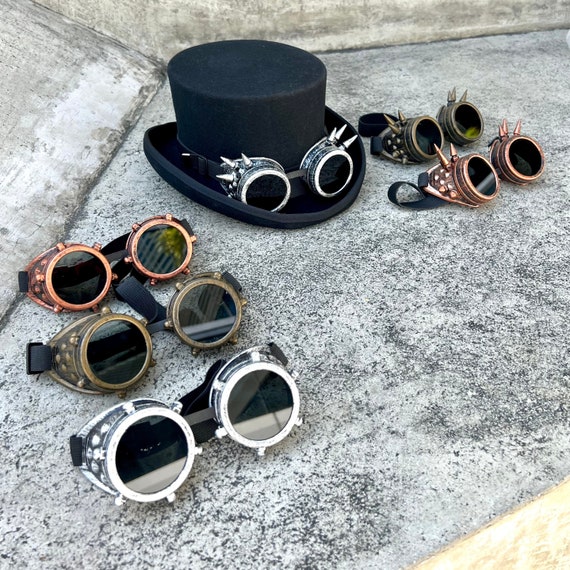This detailed photograph features a black felt top hat situated on light and dark gray concrete, accented by black discoloration and visible lines and splits. The hat is adorned with a pair of steampunk-style silver chrome goggles that are decorated with spikes, serving as a unique hat band. Positioned around the hat are five additional pairs of goggles, making a total of six. Each pair is of different metallic colors and displays the classic steampunk aesthetic. The colors include a greenish-bronze with spikes, a shiny copper with spikes, and one pair each of silver, bronze, and copper without spikes, featuring various nubs and intricate designs. All goggles have flat black lenses and black straps. The three spiked pairs of goggles are arranged to the right, while the three non-spiked pairs are on the left. The entire scene suggests a close-up view on a concrete slab, providing a detailed look at the eclectic collection of steampunk accessories.